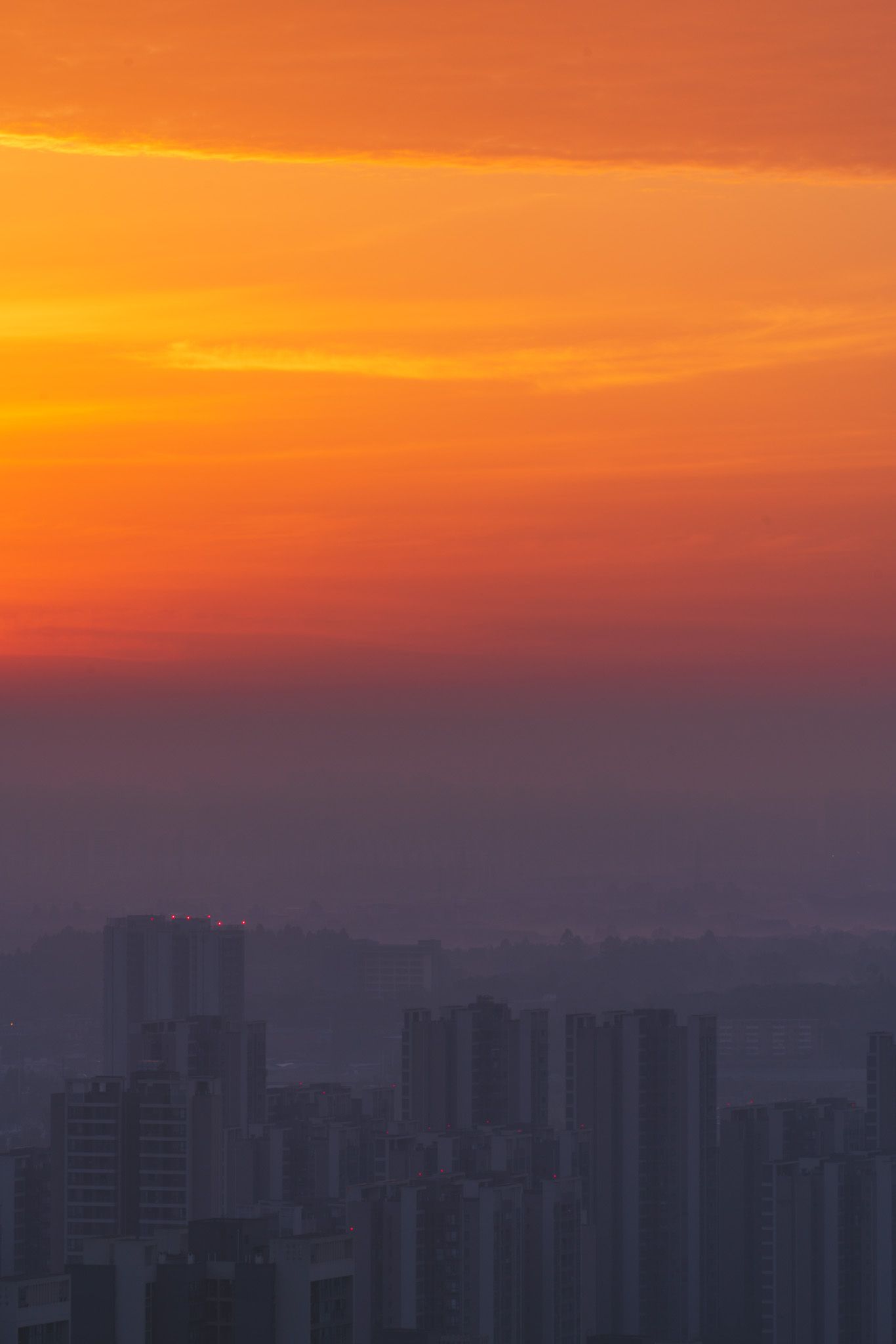The image captures a striking city skyline at sunset, shrouded in a thick layer of smog. The sky, occupying the upper half of the picture, displays a gradient of orange to deep red, interspersed with clouds that hint at the sun setting just out of view to the left. Below the vibrant sky, the scene transitions into a foggy haze that obscures the background, making it hard to discern if there are mountains or an ocean beyond the city. In the foreground, numerous high-rise buildings are silhouetted against the fading light. The buildings, possibly a mix of apartments and office towers, appear shadowy and muted, with the only notable illumination being a few red lights atop a building on the left. The pervasive smog and lack of visible activity lend an almost eerie, deserted atmosphere to the scene, suggesting an abandoned cityscape.